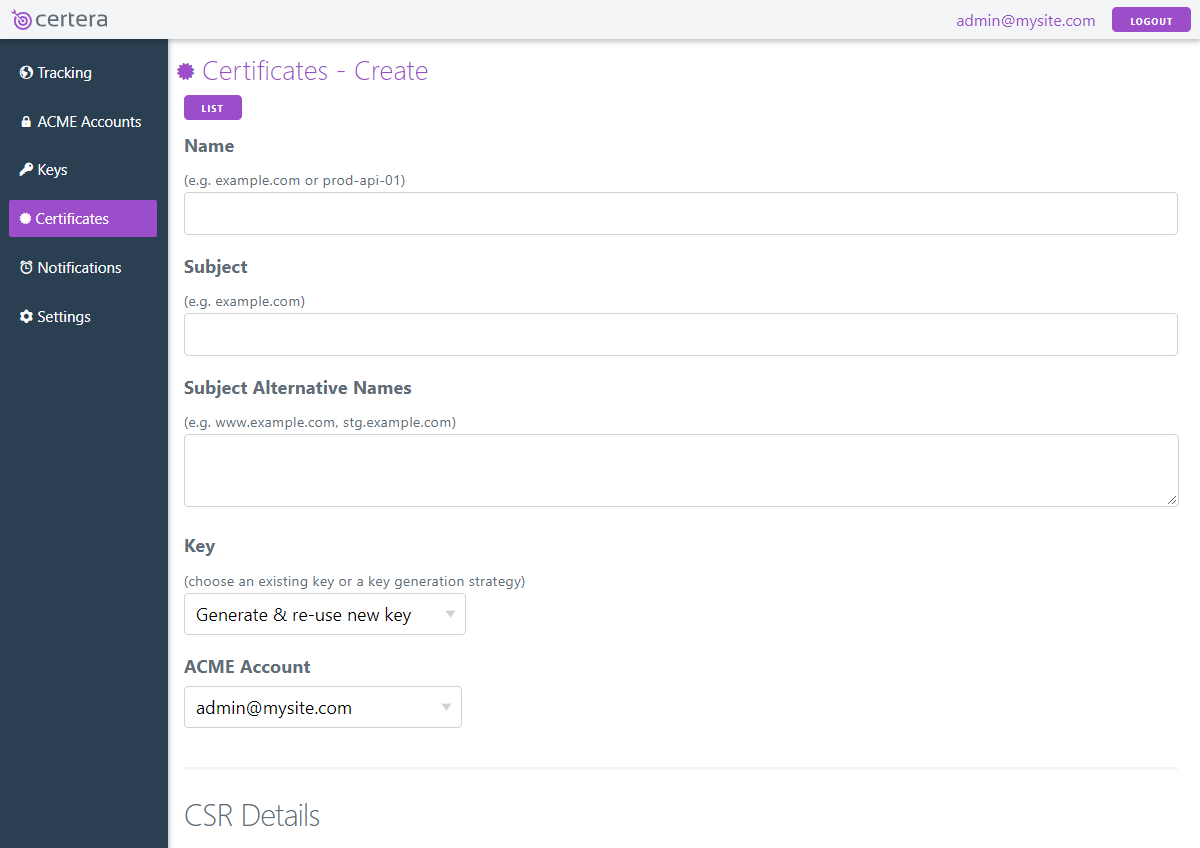The image is a color screenshot of a website for the company "certera." The company name is presented in a gray, all-lowercase font. The main logo consists of an arrow hitting a target composed of three purple concentric circles. The predominant branding colors on the page are purple, white, dark blue, and black, giving the site a functional and minimalist appearance.

The interface features a vertical navigation menu on the left side of the page with the following tabs: "Tracking," "Acme Accounts," "Key Certificates," "Notifications," and "Settings." The user has selected the "Certificates" tab, which is highlighted with a purple box, making it distinct from the other tabs that are displayed in white text on a blue background.

The main content area of the page is labeled "Certificates - Create." There is also a "List" button available. Below this heading, several fields are provided for user input, including "Name," "Subjects," "Subject Alternative Names," "Key," and "Acme Account."

The design of the webpage is straightforward and focuses on functionality, with minimal use of imagery or elaborate design elements.